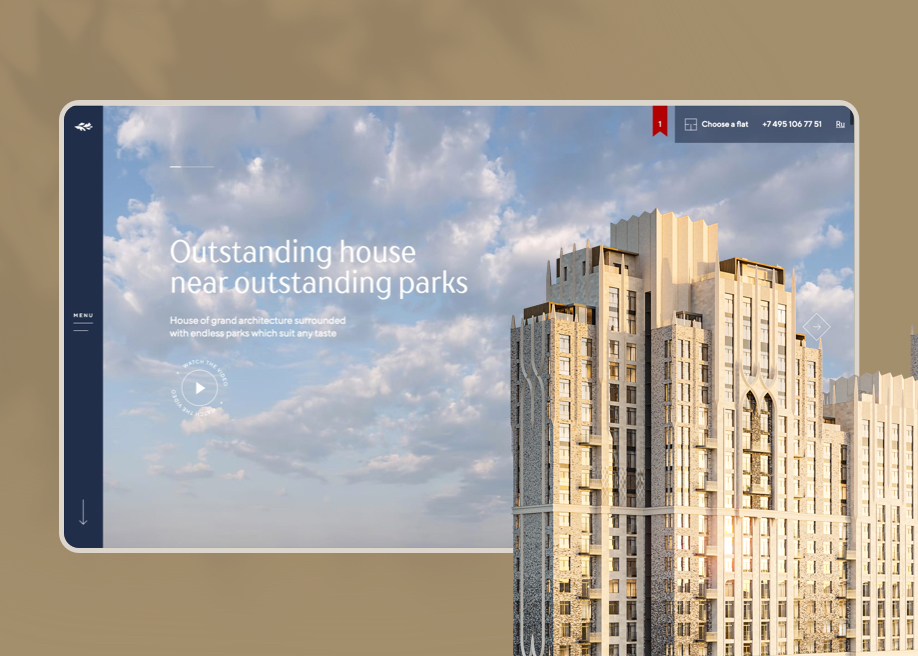The image features a gray background with a series of buildings on the right side, showcasing various levels and heights. Some of these buildings are equipped with balconies, although the majority do not have them. The backdrop behind the buildings consists of gray clouds set against a blue sky.

On the left side of the image, there is a navy blue tab labeled "Menu" with a downward-pointing arrow. Overlaying the cloud-filled background, there is a promotional text which reads: "Outstanding house near outstanding parks. House of grand architecture surrounded with endless parks, which fit any taste."

Beneath this text lies a circle with a play button icon. In the upper right corner of the image, a red ribbon hangs down. Additionally, at the top of the image on a blue background, there is a call to action that says "Choose a flat" followed by a contact number: +7495-106-7751.